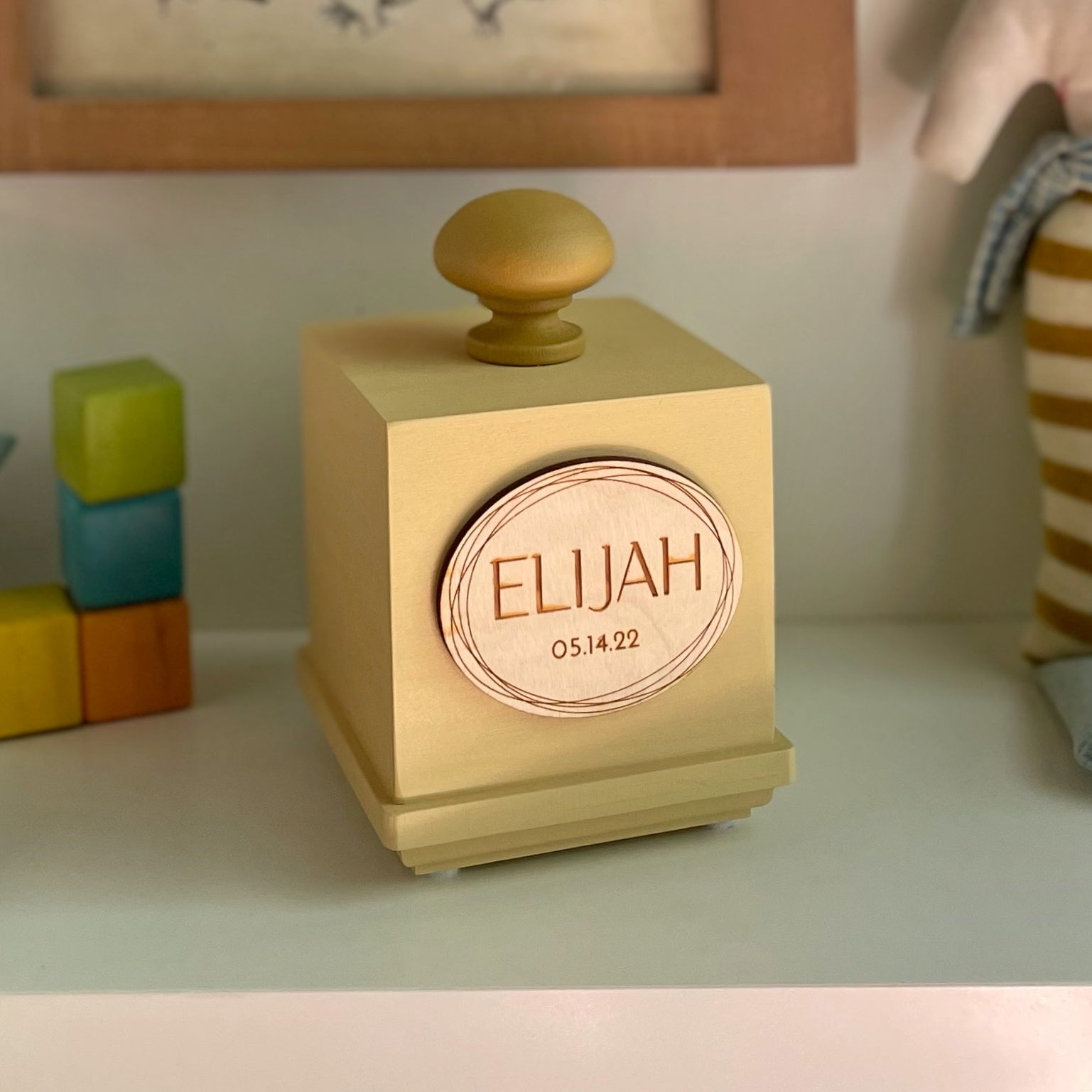The photograph depicts a nursery scene with a primarily light cream-colored aesthetic. The focus is a white wooden cube with a decorative gold knob on top, sitting on a white plastic shelf. The cube features an oval plaque on its front etched with the name "Elijah" in capital letters and the date "05-14-22." To the left of this cube, there are four stacked toy blocks in yellow, red, blue, and green, forming a reverse 'L' shape. On the right, just partially visible, is a plush toy with striped leggings, leaning against the wall and casting a shadow. Above the cube, you can see the lower part of a wooden-framed picture, though the contents of the picture are not visible. The overall composition, with its soft pastel tones and baby-themed items, suggests this is a child's room or nursery.